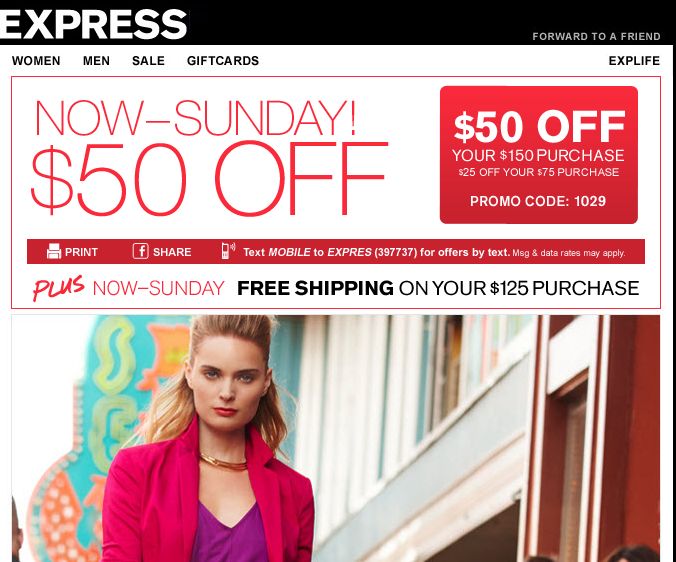This is a detailed caption for an image that captures a promotional event on the Express website:

---

Screenshot of the Express website showcasing its various categories including Women, Men, Sale, and Gift Cards tabs at the top. Prominently displayed is a large rectangular banner announcing a special offer valid through Sunday, featuring $50 off a $150 purchase and $25 off a $75 purchase with the promo code 1029. Additionally, it highlights free shipping on orders of $125 or more within the same promotional period. Users can print, share, or text the offer by messaging 'mobile' to Express to receive deals via text, with a note that message and data rates may apply.

Central to the image is a stylish woman modeling in a vibrant downtown setting. She wears a purple top, possibly a dress, complemented by a gold necklace and a striking pink jacket. Her hair is styled half-up and half-down, adding to her poised and confident look. She gazes directly into the camera, creating a captivating focal point. Though there are other people around her, they are just out of full view, their presence hinted by the tops and sides of their heads. The bustling urban background enhances the dynamic and trendy atmosphere of the scene.